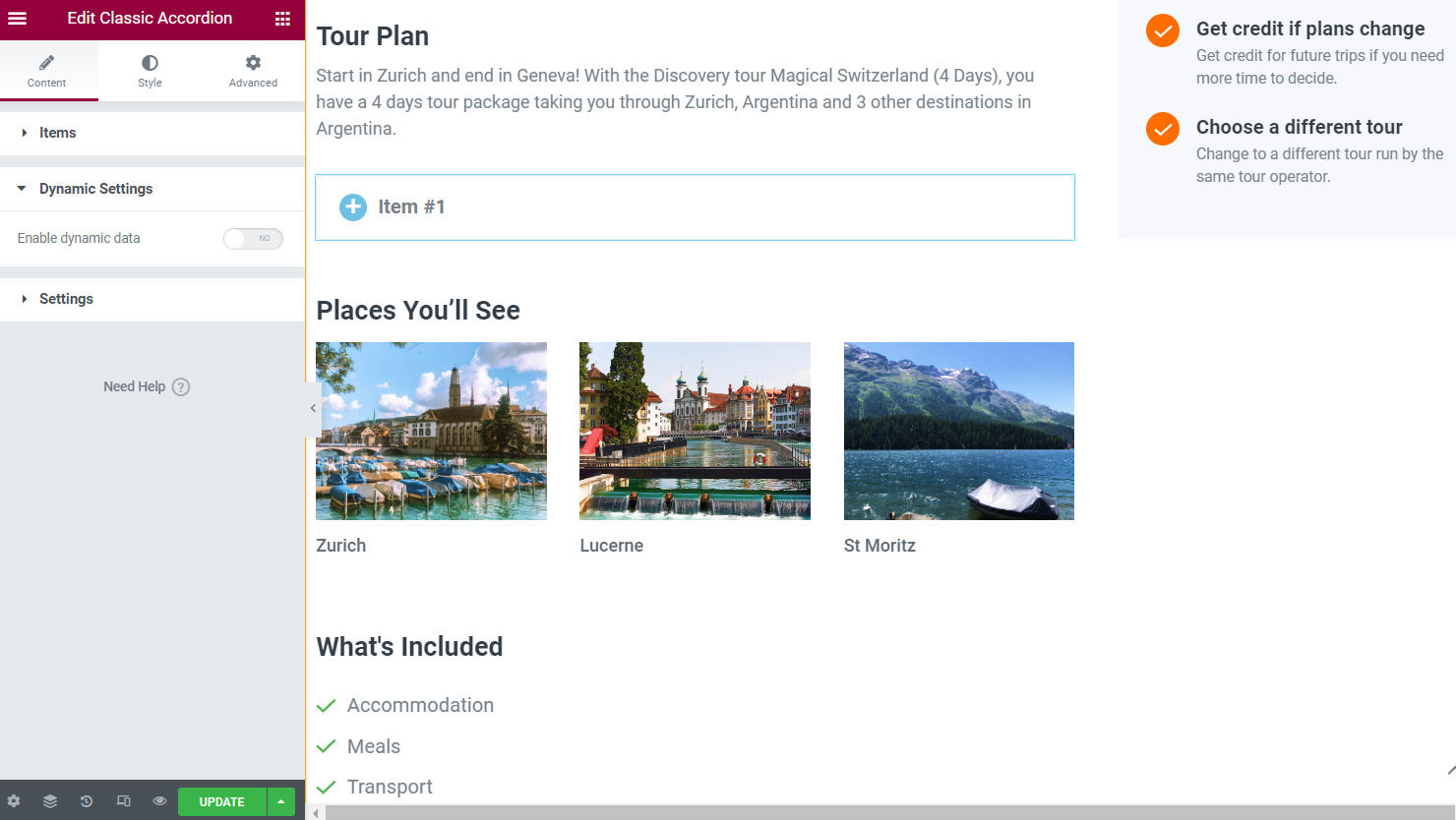**Holiday Brochure Page: Tour Plan Overview**

This is a detailed brochure page from a holiday tour showcasing the "Magical Switzerland" four-day discovery tour. The top section of the page introduces the journey, which begins in Zurich and concludes in Geneva. This itinerary is part of a four-day tour package that covers Zurich, Lucerne, St. Moritz, and other notable Swiss destinations.

On the right-hand side, there are several headings with orange circles and ticks indicating various options and assurances available for travelers:
- "Get Accredited Plans"
- "Change and Choose a Different Tour"

Beneath the tour plan summary, the brochure provides a brief visual tour with images of key destinations:

1. **Zurich**: The first image captures a large building in Zurich, set against a picturesque marina with boats docked.
2. **Lucerne**: The second image features Lucerne, showcasing serene waters with a majestic chateau in the backdrop.
3. **St. Moritz**: The third picture highlights St. Moritz, with its stunning mountain scenery, a tranquil lake, and what appears to be a cabin in the foreground.

The inclusions section outlines the essentials covered in the tour:
- Accommodation
- Meals
- Transport

However, only a partial view of this section is visible in the brochure, indicating that additional details might be available on the full page.